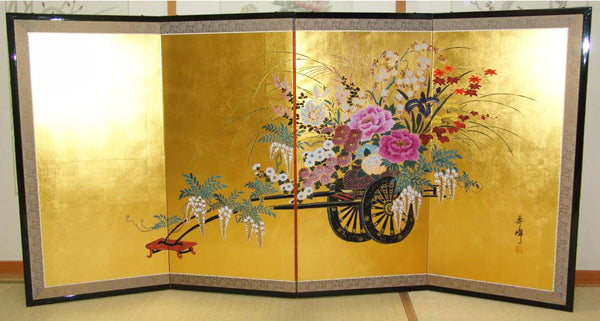The photo captures a traditional Japanese folding screen consisting of four segments, each bordered by a gray and black frame. The background of the screen is a vibrant gold, adorned with an intricate depiction of a hand cart or rickshaw brimming with an array of colorful flowers and foliage. The cart, which has two large wheels and is seemingly floating on the golden panels, is piled high with flowers in shades of orange, yellow, purple, pink, white, and red, along with green ferns and leaves. The screen itself is positioned against a white, subtly patterned wall, reminiscent of a traditional Japanese house with tatami mats on the floor and a distinct piece of wood running underneath. The scene evokes the aesthetic of Japanese art and craftsmanship, portraying a market-bound floral cart in a beautifully ornate setting.